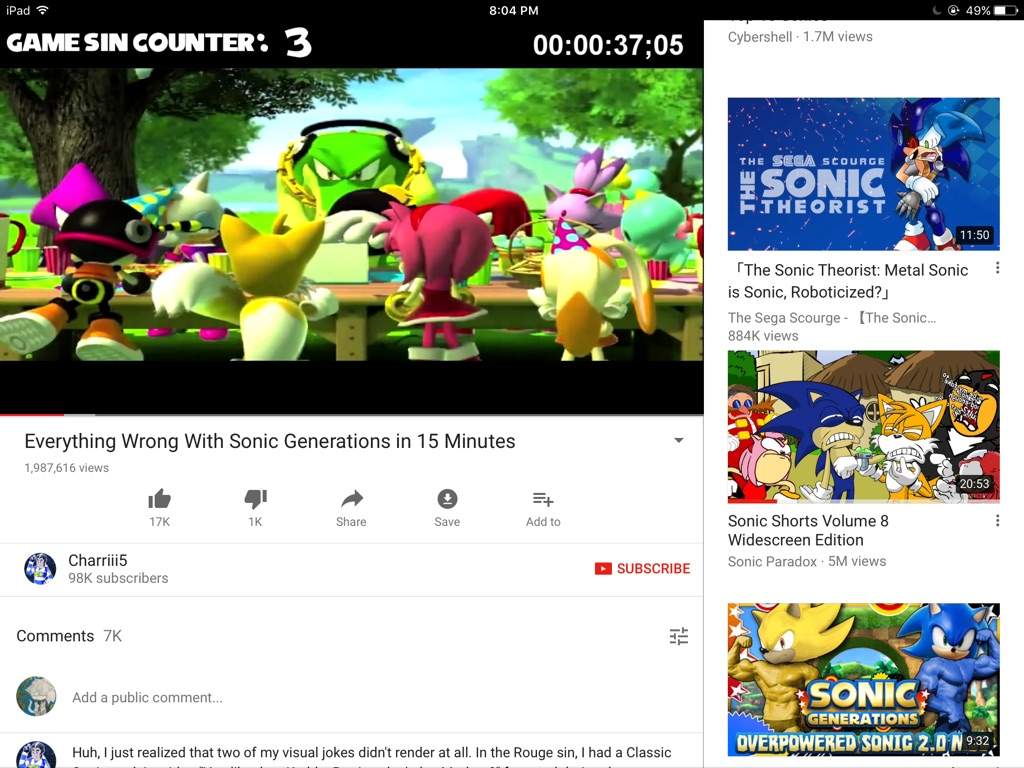The image displays a YouTube app interface on an iPad tablet. In the top left corner, the iPad label and Wi-Fi symbol are visible. The top center displays the time at 8:04 p.m., while the top right shows the battery is at 49% and the device is locked from auto-rotating.

The YouTube Play window on the left side features a video titled "Everything Wrong With Sonic Generations in 15 Minutes." The video is paused at 37:05, showcasing game characters including Tails from Sonic the Hedgehog in a forest-like setting, where they appear to be feasting at a table. The video has garnered 1.9 million views, 17,000 likes, and 1,000 dislikes, indicating that it was uploaded before YouTube started hiding dislike counts. 

The channel "Chari5" is identified as the content creator, boasting 98,000 subscribers. A red subscribe button is visible alongside the show's engagement statistics, revealing 7,000 comments. To the right, a list of recommended videos is displayed in a vertical strip.